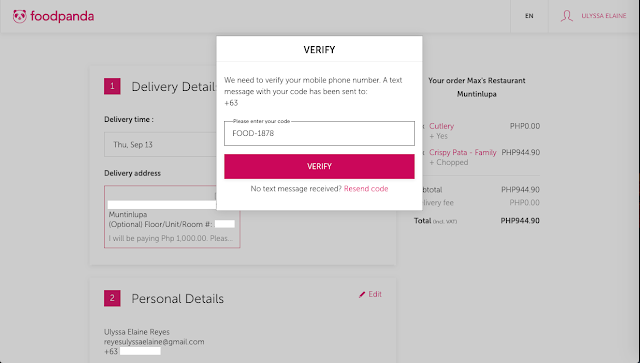This is a detailed description of an image of the Foodpanda website:

At the top left corner of the image, the recognizable face of a panda logo appears, immediately followed by the word "Foodpanda" highlighted in a purplish hue. On the top right corner, the abbreviation "EN", indicating the English language, is displayed, separated by a vertical line. Adjacent to this is an icon of an unidentified person, accompanied by some blurred text that is not discernible.

Centrally positioned on the webpage is an overlapping verification box with a message instructing the user to verify their mobile number. It reads: "We need to verify your mobile number. A text message with your code has been sent to +63." Below this message is a text box containing a placeholder code "food-1878". Underneath this, a long rectangular button labeled "Verify" is prominently displayed. Following this, the text "No text message received?" is presented with a "Resend Code" option highlighted in the same purple color.

Below the verification box, partially obscured, is another section with two labeled steps: "1. Delivery details" and "2. Personal details". Some of the information in this section is whited out for privacy, including fields related to delivery details and a phone number.